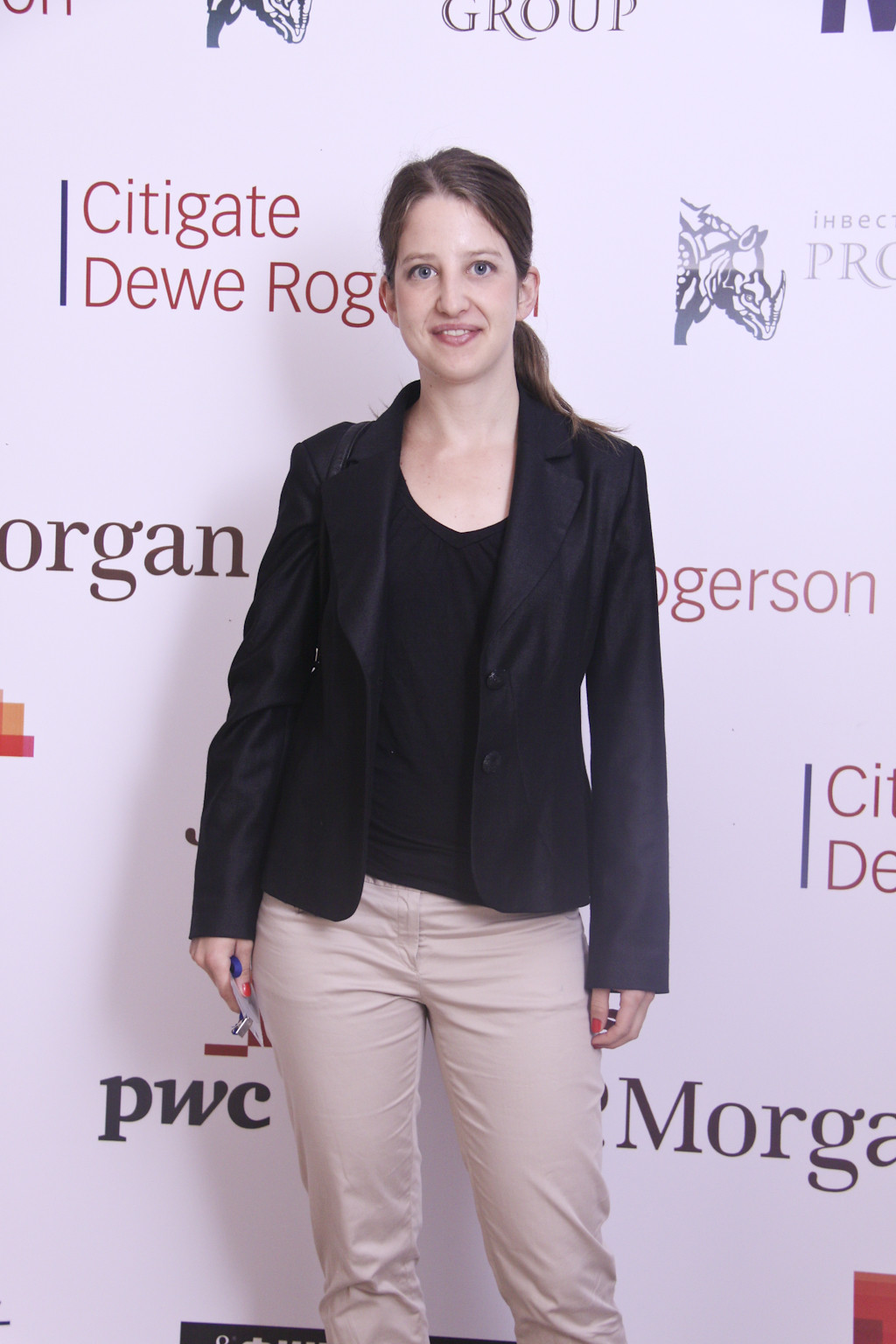In the photograph, a young woman in her twenties is captured standing in front of a sponsor-laden event backdrop. Her long brown hair is neatly pulled back into a ponytail. She is dressed in a blue blazer over a black v-neck top, paired with beige or light brown pants. Her attire appears to be business casual, and she has a bag strap slung over her left shoulder, with something clutched in her left hand. The woman, with gray eyes, attempts a smile that borders on a grimace. Behind her, the backdrop features logos and names of various sponsors, including Morgan Stanley, JP Morgan, PWC, Citygate, Dewey, Rogerson, and a graphic of a rhinoceros. The image is portrait-oriented, taller than it is wide.